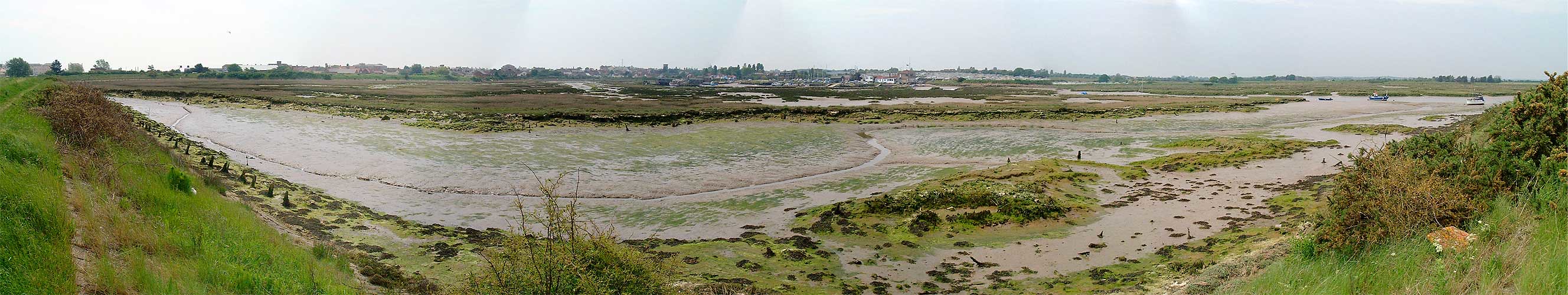This photograph captures a long panoramic view of a marshy, swampland landscape. Dominated by a central body of muddy water that curves and rounds towards the front and back, the scene features a mixture of sandy and muddy areas creating a shiny, beige, brown, and greenish surface. At the edges, you can see patches of green grass, some of which appear to be browning or drying out, interspersed with bushes and sloping terrain. The backdrop showcases a flat expanse of green land under a sky that transitions from really light blue at the top to a dusty appearance with heavy clouds, devoid of visible sunlight. The panoramic layout presents the landscape in a concave, circular form, enhancing the viewer's sense of immersion in this natural, yet somewhat desolate setting.